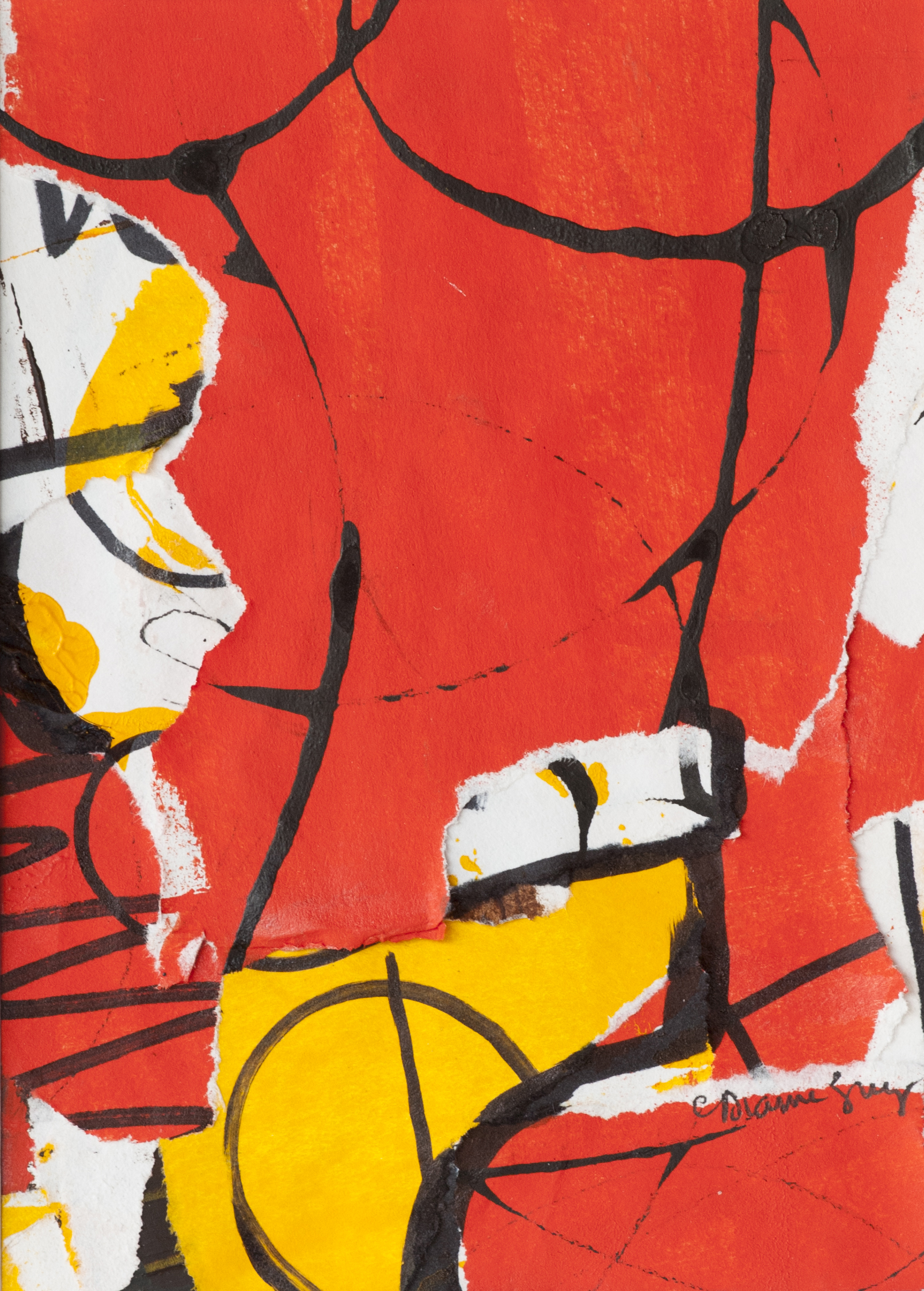The image features a tall, rectangular mural set on public ground, predominantly painted in vibrant red hues. The mural, an abstract art piece, showcases a dynamic composition with black curved and streaking lines, along with splotches of primary yellow and stark white. These elements create an intricate pattern of vertical and horizontal lines, circles, and squiggles, contributing to its busy and interpretative nature. Notably, at the bottom right corner, there is a watermark signature by the artist, Diane Song or Diane Gray. The entire mural is vividly colored, with emphasis on bold reds accented by black, yellow, and white, making it a striking and engaging artwork open to viewers' interpretation.